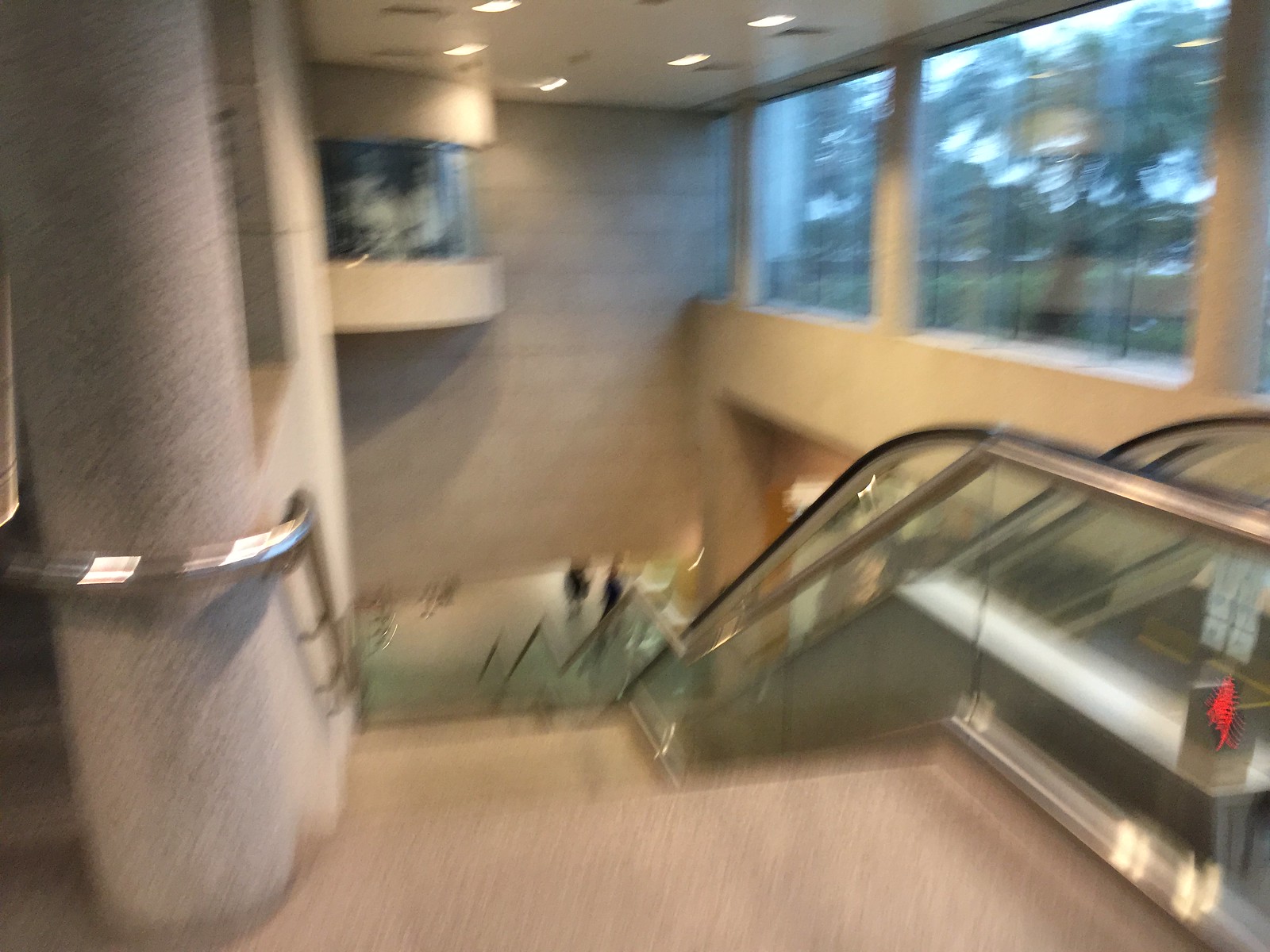The image captures a downward perspective of an escalator integrated into a staircase, likely taken in a bustling venue such as a mall, airport, or large entertainment complex. The shot is angled obliquely, giving a 'kitty-corner' view across both the stairs and the escalator. The flooring and walls feature a light tan carpet with subtle hints of mauve or pink, extending up the lower portions of the walls. The overall scene has a slight blur, suggesting the photo was snapped while in motion, and is under soft lighting, adding to the subdued atmosphere. At the base of the escalator, a few individuals stand idly, reinforcing the likelihood of a transitional space like an airport. The right-hand wall is lined with windows, revealing a view of lush, blooming vegetation outside under an overcast sky, with indications of potential rainfall.